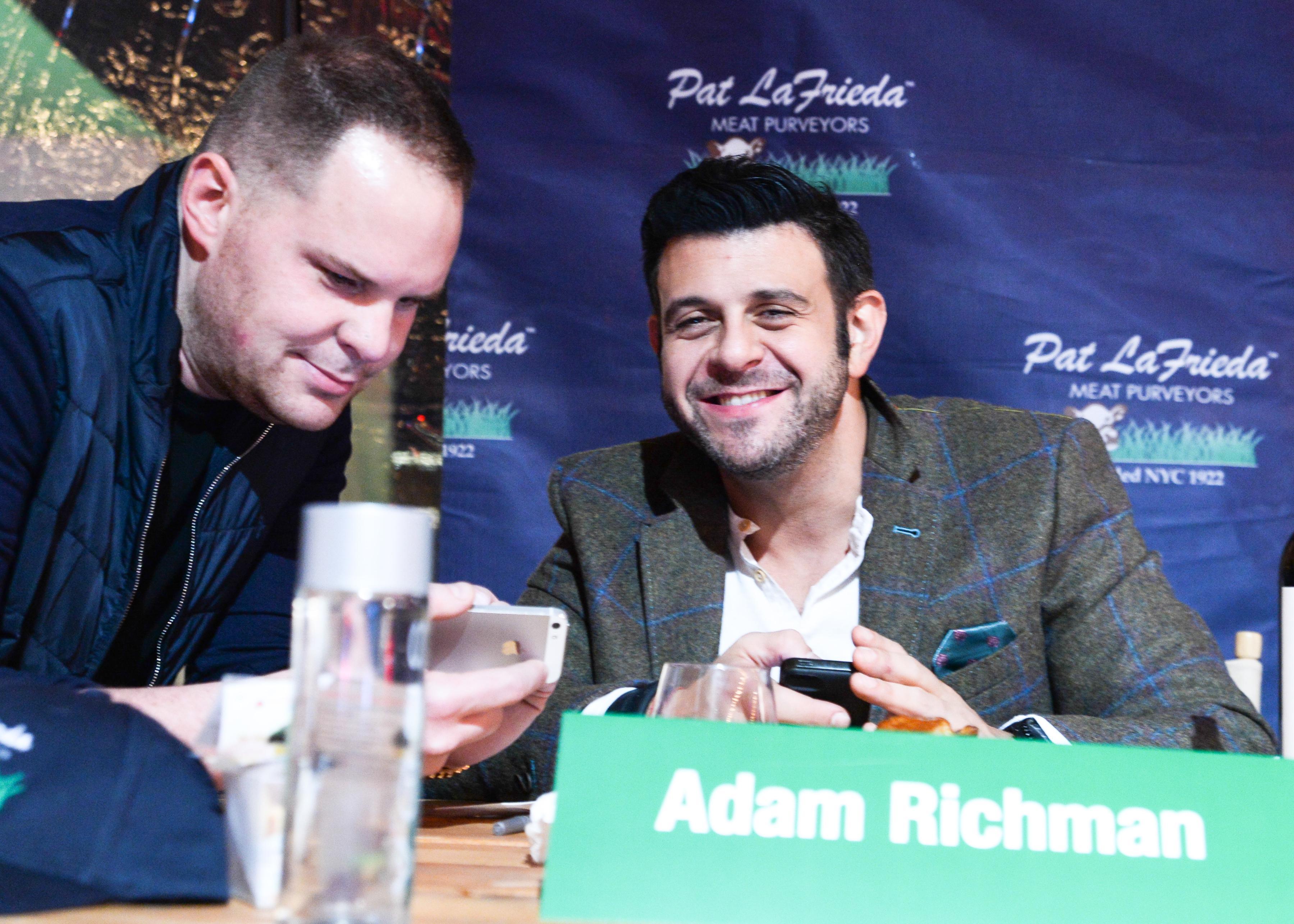In this detailed color photograph, we see two men interacting closely. The central figure, identified by an aqua-colored placard with bold white letters as "Adam Richman," sits at a table. He has dark hair, a scruffy mustache, and beard, and he is smiling broadly, displaying his teeth. Adam wears a gray blazer adorned with a blue grid pattern, a white shirt, and a blue pocket kerchief. His arms are propped up on the table, holding a cell phone in his hands. To his left, another man, likely a fan, is leaning over towards Adam, engrossed in his cell phone. This man has short, dark hair and is dressed in a dark jacket over a blue quilted vest. The background features a blue banner with the repeated logo "Pat LaFrieda Meat Purveyors," accompanied by green and gold accents. A bottle of water with a gray cap sits on the left side of the table, adding to the scene's authenticity and casual tone. The image captures a moment of interaction, presenting a sense of realism and representational detail.